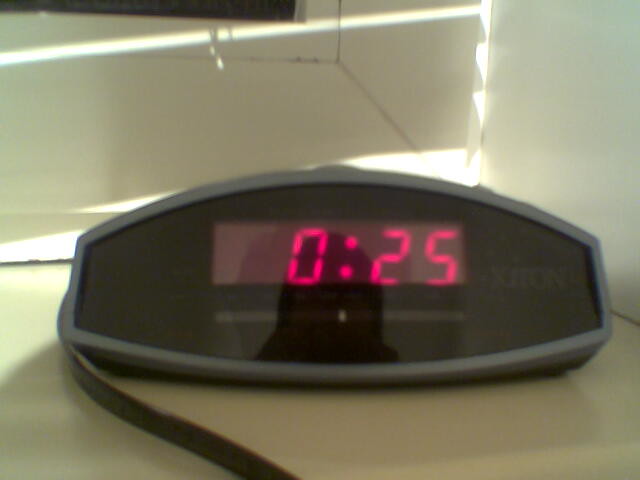This intimate photograph showcases a close-up view of a device, possibly an alarm clock or a medical apparatus. The device prominently displays a name on its side, which appears to be "XIRON." The device features a sleek black face with bright red digital numbers, reminiscent of an alarm clock's display. Its outer casing is a unique grayish-purple hue. Despite the photo's slight blurriness, the device is clearly resting on a cream-colored tabletop. The background walls are stark white, enhancing the contrast in the image. Upon closer inspection, a reflection can be seen on the device's surface, revealing the silhouette of the photographer who seems to be wearing a hood, partially obscuring their features. The overall composition offers a sense of curiosity and intrigue, drawing attention to the mysterious device and its environment.